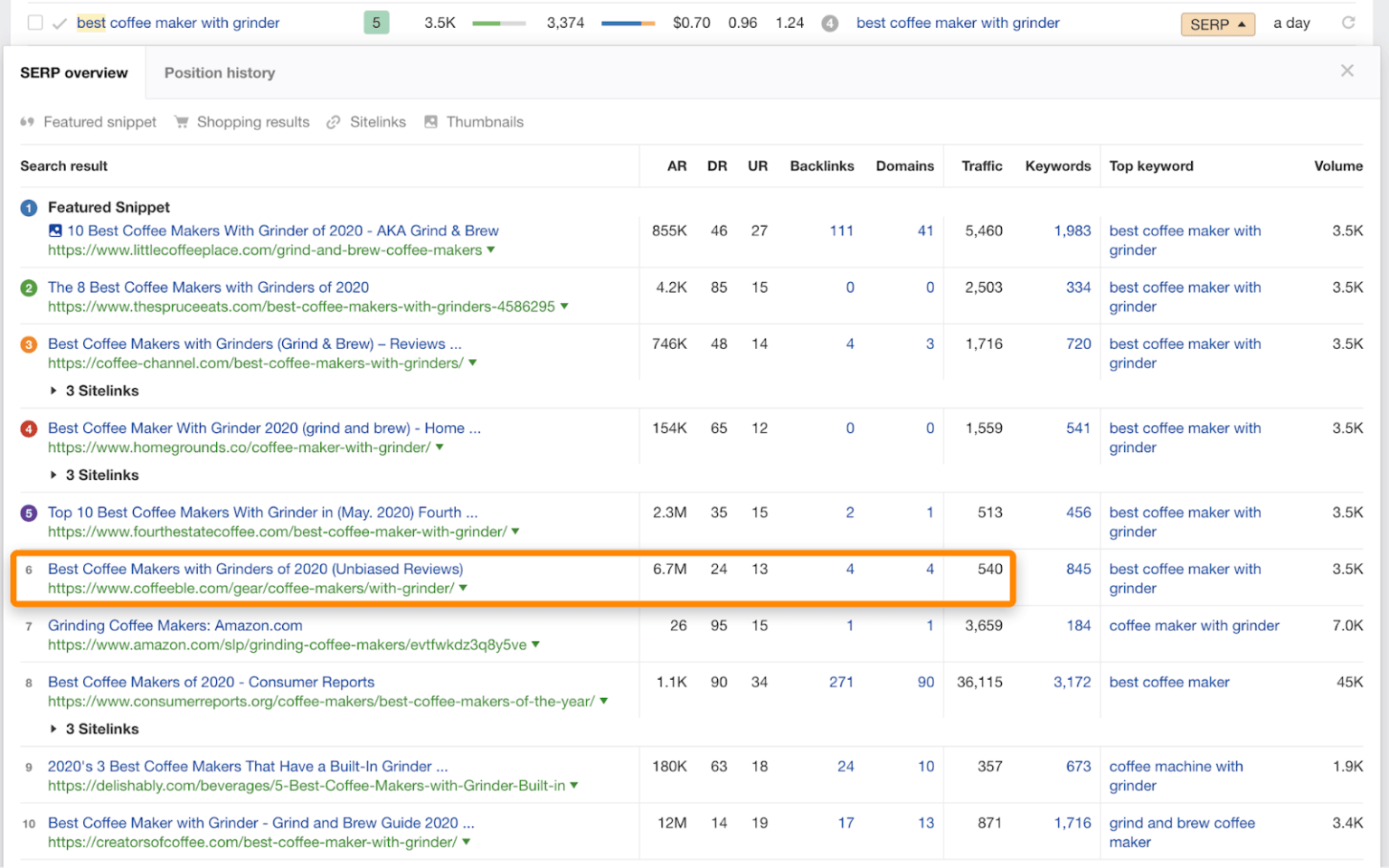The image is a detailed screenshot of a search result analysis table for the query "best coffee maker with grinder," with the word "best" highlighted in yellow. At the top of the table, there are two tabs: "SERP Review" and "Position History," with "SERP Review" currently selected.

Underneath, the search results are displayed, starting with a featured snippet titled "10 Best Coffee Makers with Grinder 2020 (aka Grind and Brew)." The subsequent search results are listed as follows:
1. "The 8 Best Coffee Makers with Grinders of 2020"
2. "Best Coffee Makers with Grinders (Grind and Brew Reviews)"
3. "Best Coffee Maker Grinder 2020 (Grind and Brew Home)"
4. "Top 10 Best Coffee Makers with Grinder May 2020..."
5. "Best Coffee Makers with Grinders of 2020 (Unbiased Reviews)" – this entry is highlighted with an orange box.
6. "Grinding Coffee Makers: Amazon.com"
7. "8 Best Coffee Makers of 2020 (Consumer Reports)"
8. "2020 Best Coffee Makers with Built-in Grinder"
9. "Best Coffee Maker with Grinder (Grind and Brew Guide 2020)"

The table includes various metrics for each result, such as AR, DR, UR, backlinks, domains, traffic, keywords, top keywords, and volume, all filled in with their respective numbers, providing comprehensive SEO data for the listed websites.